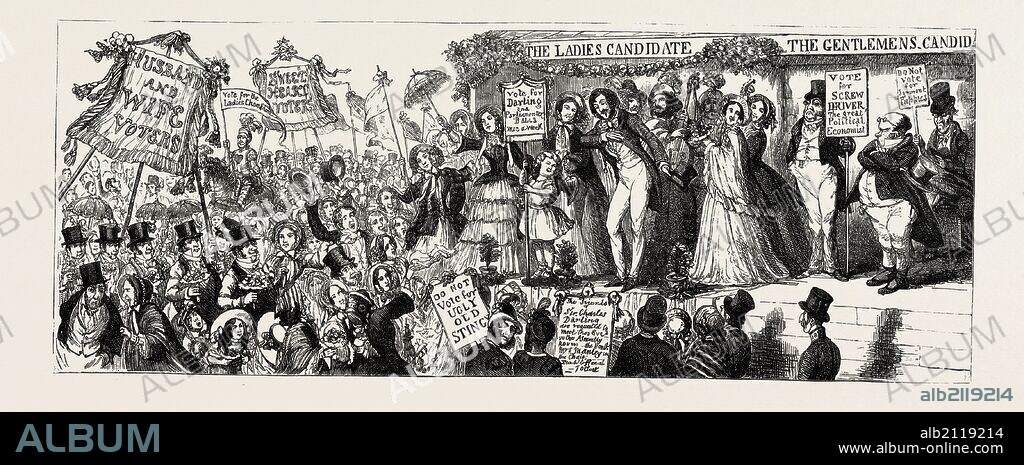This detailed hand-drawn illustration, done in a black and white, pencil or charcoal style, captures a Victorian-era scene focused on women's suffrage. The rectangular image prominently features a stage with a banner in the background, reading "The Ladies' Candidate" and "The Gentlemen's Candidate." Center stage is a man in a petticoat with white pants, bowing with his hat in his left hand. To his right stands a woman in a dress, bonnet, and jacket, accompanied by a small child. Several other men and women on the stage hold signs endorsing various candidates. In the audience below, a diverse group of men and women, some in black top hats, hoist signs, including one that reads, "Do Not Vote for the Ugly Old Stingy." Another prominent sign reads, "Husband and Wife Voters." The image also features a knight on horseback in the background, adding a historical flair. The lower left corner contains the text "album," while the lower right corner features the website "www.albumonline.com."